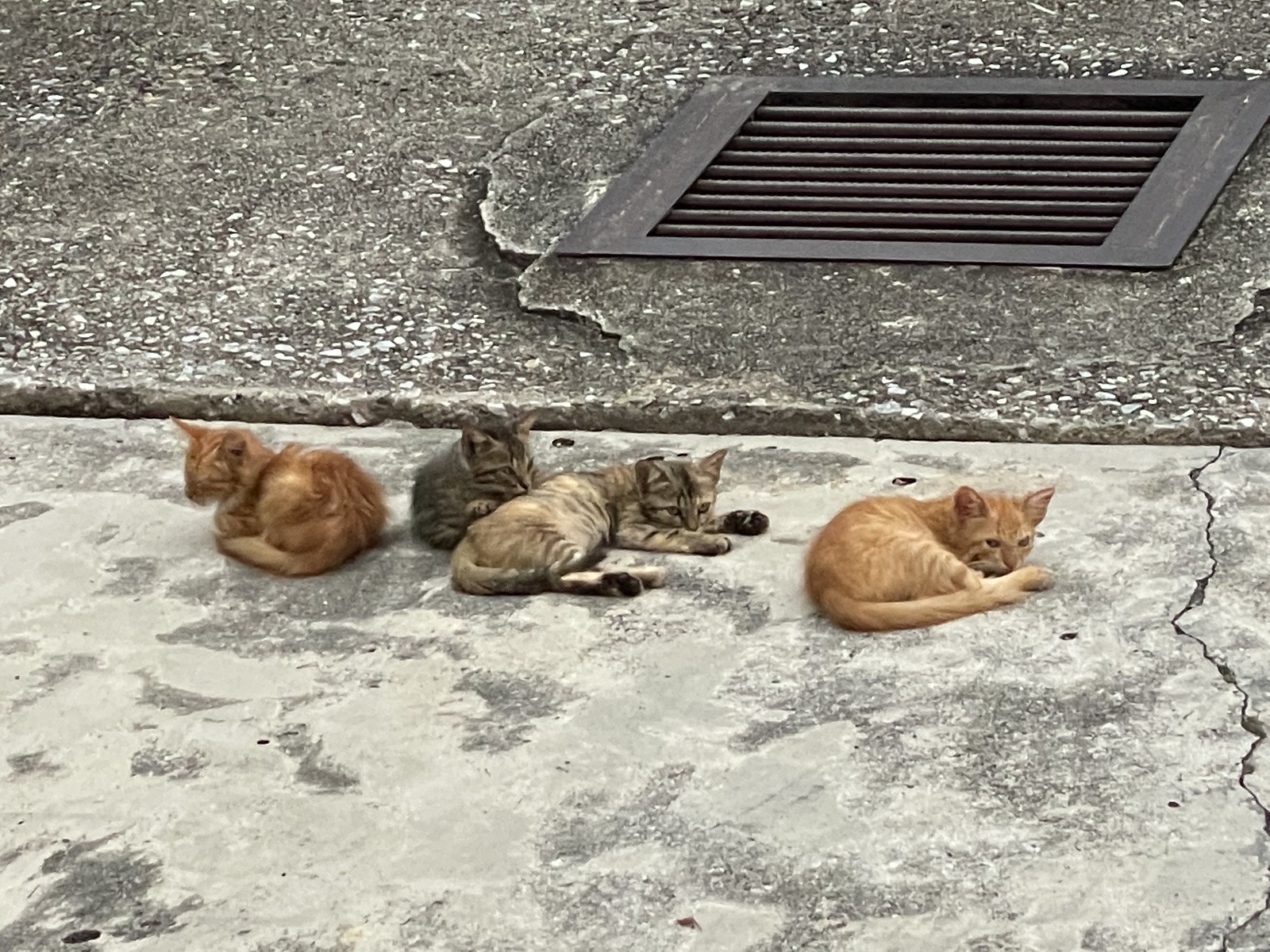This is a color photograph of four seemingly stray cats lying or sitting on a light grey pavement scattered with darker grey shingles. All cats appear to be mature and a bit scruffy. From left to right, there is an orange tabby cat facing left, a nearly black striped cat, and a cream and lighter striped cat, both of which are in the middle, facing slightly to the right, and appear to be lying on each other. On the far right, there is another orange tabby curled up on the ground, facing right. Behind the cats is a rougher, darker grey concrete area that looks more shingly, and near the upper right corner, there's a lopsided, rectangular street vent or grid with a noticeable squiggly crack underneath it. The setting suggests an outdoor urban environment with visible details of cracks and weathered asphalt.